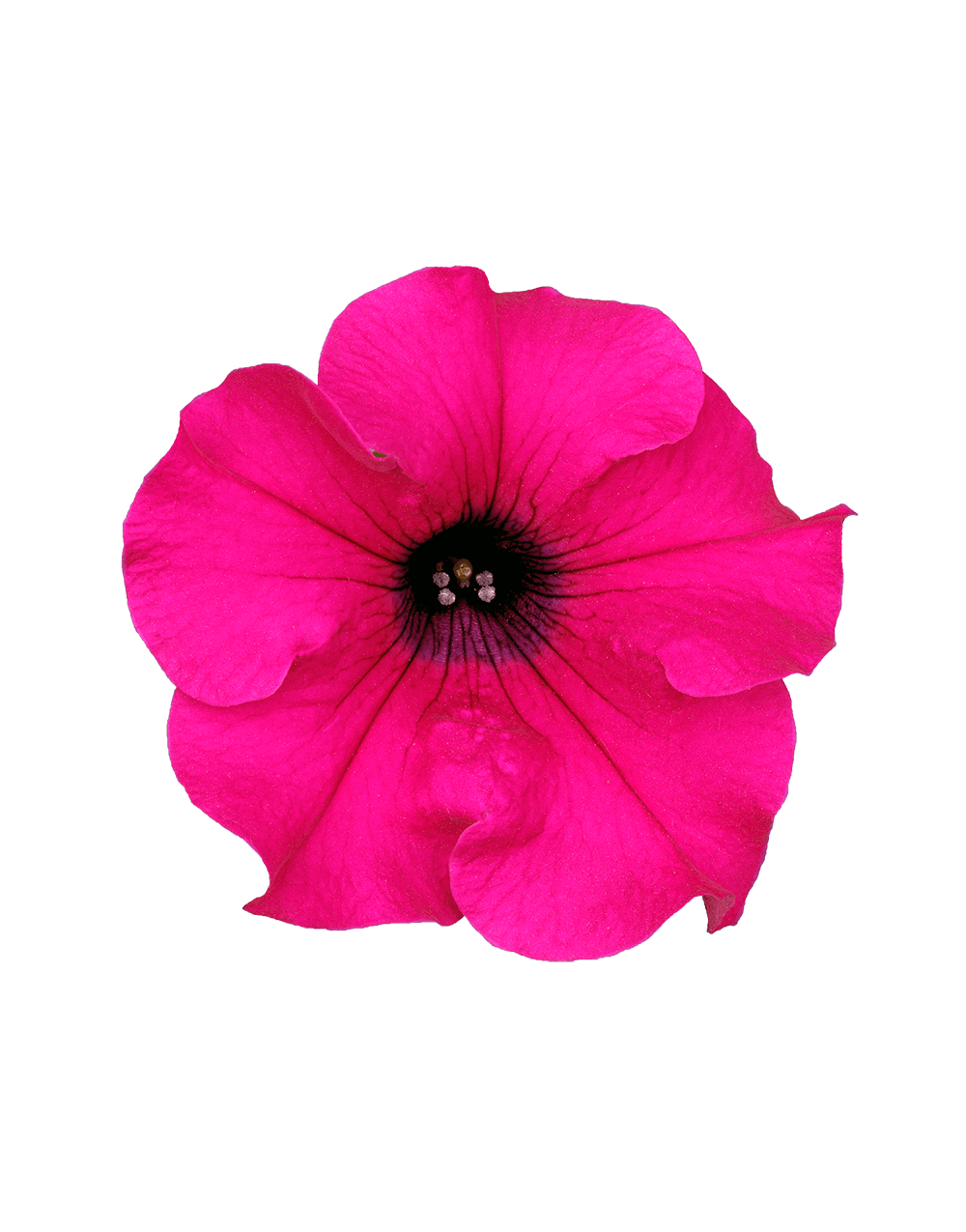The image is a detailed, close-up view of a single hot pink flower, likely a hibiscus or possibly an orchid, set against a stark white background. The photograph captures only the vibrant petals and the intricate interior, omitting any stem. The petals radiate delicate shades of fuchsia and hot pink, transitioning to a darker, burgundy-ish pink as they approach the center. 

The heart of the flower reveals a striking contrast with a dark, nearly black center speckled with very small white seeds or pollen. Fine lines extend outward from this central area, emphasizing the delicate structure of the petals. The position of the flower is front-facing, as the perspective offers a bird's eye view, focusing on the exquisite details of the flower's coloration and texture against a simple, unadorned background.